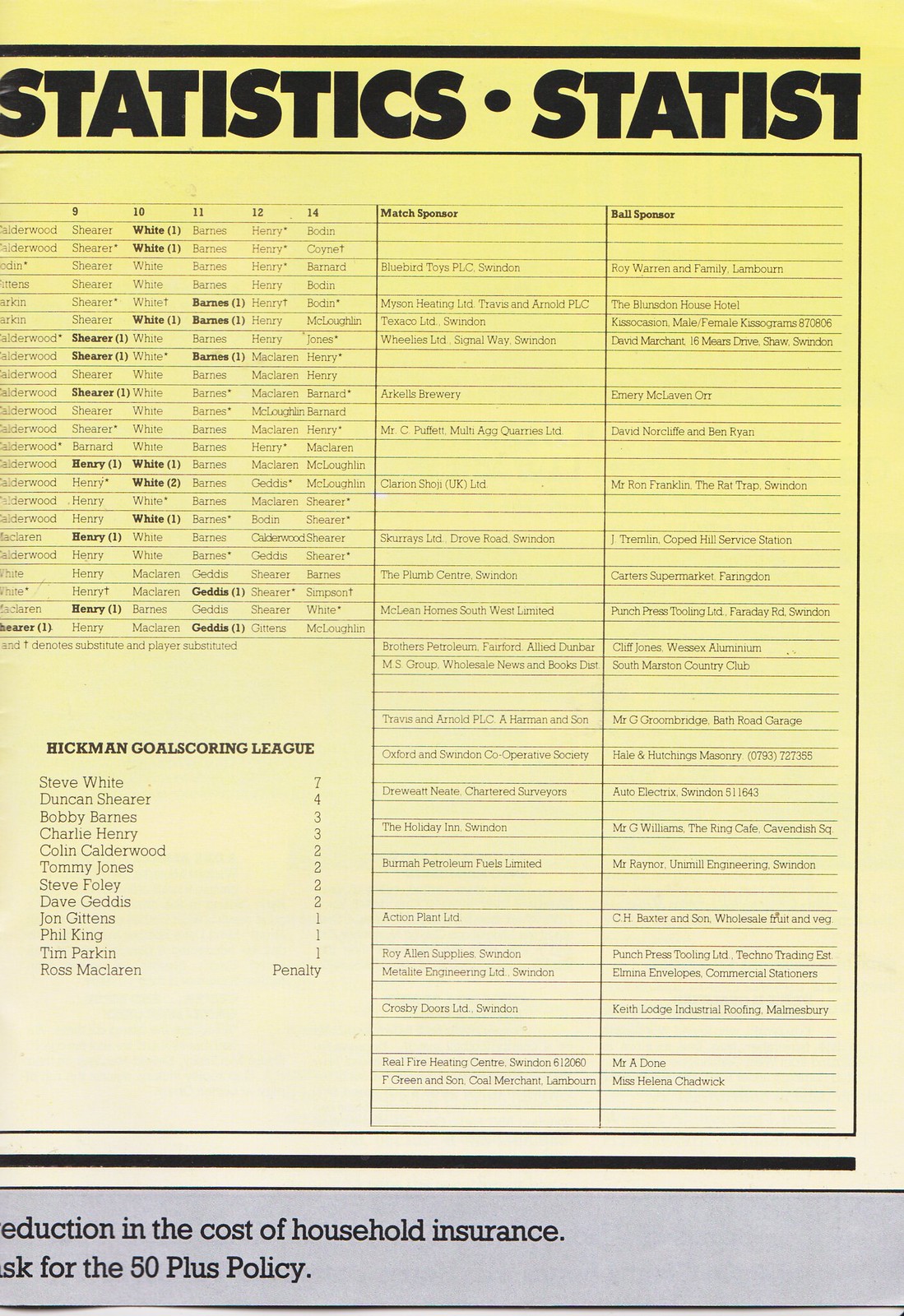This image depicts a vertical, rectangular statistics sheet with a dull yellow background and black text. The header prominently reads "Statistics," although the exact wording appears repetitively and some parts are cut off. The layout is organized into several columns with tiny, hard-to-read text and numbers, including 9, 10, 11, 12, and 14, which are positioned in rows on the left.

Prominently in the lower left section, the title "Hickman Goalscoring League" is clearly visible. Below this title, the sheet lists various players along with the number of goals they have scored: Steve White leading with 7 goals; Duncan Shearer with 4; Bobby Barnes and Charlie Henry both with 3; Cullen Calderwood, Tommy Jones, and Stephen Foley each with 2; Dave Geddes, John Gittens, and Phil King all with 1 goal; and Ross McLaren noted with a penalty.

Additionally, the sheet includes sections marked "Sponsor" and "Ball Sponsor" with their respective information in columns. The bottom part of the sheet hints at an advertisement related to health insurance, specifically mentioning a reduction in the cost for the 50-plus policy. The predominant colors of the document are yellow, white, and light gray.